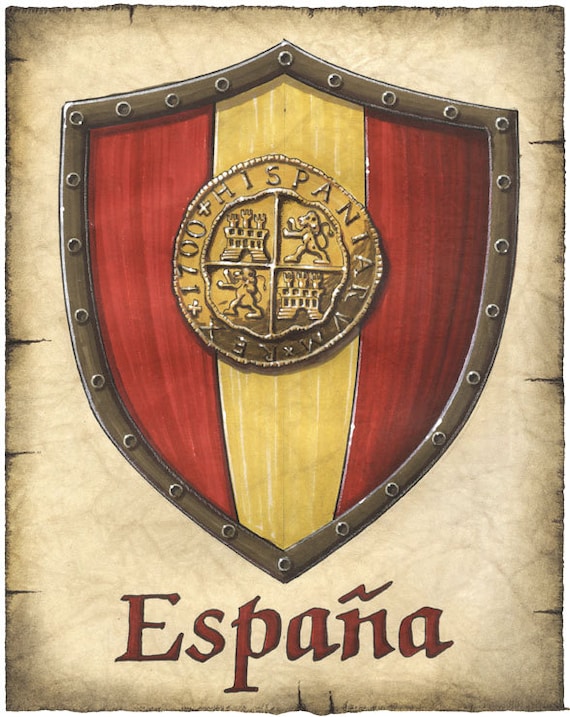This digital artwork, resembling an old poster, features a prominently displayed coat of arms at its center. The artwork has a nostalgic feel, achieved by a tan background designed to mimic old, torn parchment paper with rips along its edges. At the core of the image is a shield, made to look brass, divided into three vertical sections: the left and right sections are a dark red maroon color, while the center section is a golden yellow. Intricately detailed within a circular seal overlaying the golden section are depictions of a standing lion and a castle, among other elements. Below the shield, the word "España" is inscribed in dark red lettering, matching the color of the outer sections of the shield, enhancing the coat of arms' regal appearance. The entire composition has a cartoon-like style, augmenting its artistic charm.